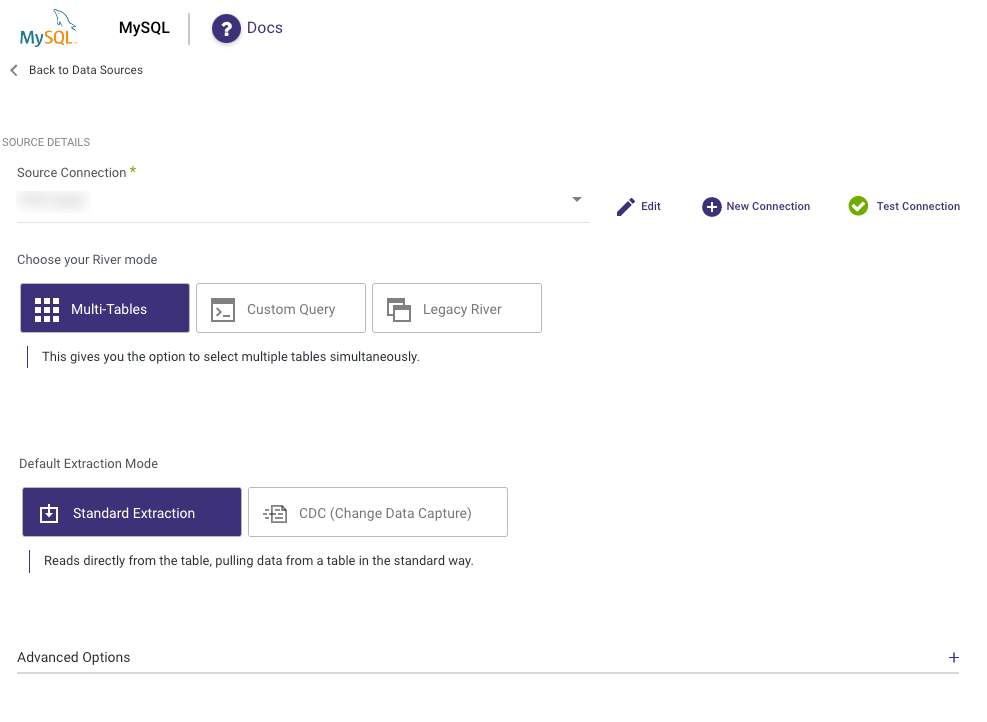This image is a screenshot from the MySQL website, specifically showcasing the data source connection setup page. In the upper-left corner, the MySQL logo featuring a dolphin is displayed prominently. Just to the right of the logo, the word "MySQL" is written, followed by a blue circle with a white question mark in its center, indicating a help or documentation section labeled "docs." 

Below this header, there is a navigational link labeled "Back to Data Sources" accompanied by a left-pointing arrow, which allows users to return to the previous page.

The main content area of the page details the source connections. It features a section titled "Source Connection," marked with an asterisk indicating a required field. Below this, there is a drop-down form field for selecting multiple options. Adjacent to the drop-down, there are three buttons labeled "Edit," "New Connection," and "Test Connection" for managing and verifying database connections.

Further down the webpage, there are two prominent sections. The first is "Choose Your River Mode," with a highlighted blue button labeled "Multiple Tables." The second section is "Default Extraction Mode," featuring another blue button marked "Standard Extraction."

The final element on the page is an "Advanced Options" field, which includes a plus sign on the far right. This suggests the availability of additional options that can be expanded or accessed via another page.